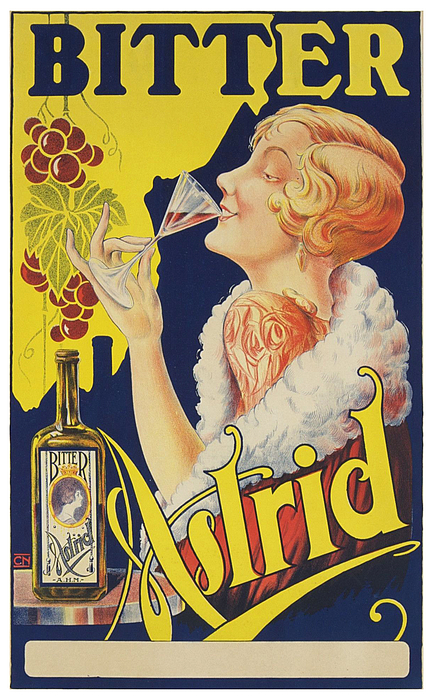The poster is a vintage-style advertisement, likely from the 1920s, featuring a flapper woman in the center. She has blonde, bobbed hair and is dressed elegantly in a red robe, complemented by a luxurious white fur stole draped over her shoulders. Facing left, she holds a cosmopolitan-style glass delicately, sipping with her pinky and ring finger raised. The background is primarily dark blue, transitioning to yellow at the top, decorated with clusters of grapes and leaves.

The word "Bitter" is prominently displayed at the top, split between blue letters over the yellow section and yellow letters over the blue section. The word "Astrid" is written in cursive on the bottom right, accentuated with decorative flourishes. On the bottom left, there is a bottle of a beverage labeled "Bitter Astrid," which features a headshot of the woman from the poster. The entire image is brightly lit and vividly colored, highlighting the clarity and details of the advertisement.